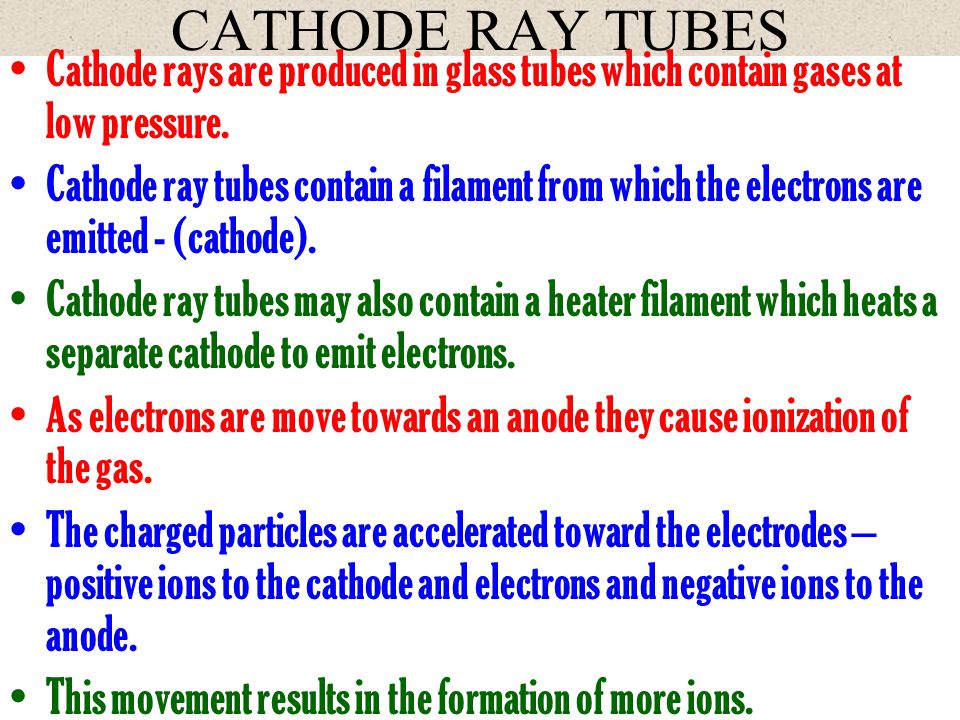The image appears to be a PowerPoint slide with a white background, featuring a detailed description of Cathode Ray Tubes. At the very top, there is a large beige rectangle spanning the entire width of the image. In the center of this rectangle, in black, serif font and all capital letters, it reads "CATHODE RAY TUBES."

Below this headline, there is a series of bullet points, each in different colors. The first bullet point, in red, states: "Cathode Ray Tubes are produced in glass tubes which contain gases at low pressure." The next bullet point, in blue, explains: "Cathode Ray Tubes contain a filament from which the electrons are emitted (cathode)." Following this, a green bullet point elaborates: "Cathode Ray Tubes may also contain a heater filament, which heats a separate cathode to emit electrons." Another red bullet point notes: "As electrons are moved towards an anode, they cause ionization of the gas." Following in blue, it says: "The charged particles are accelerated toward the electrodes, positive ions to the cathode, and electrons and negative ions to the anode." The final green bullet point concludes: "This movement results in the formation of more ions."

Overall, the image is a clear and structured presentation of how Cathode Ray Tubes function, with multicolored text enhancing readability and emphasizing key points.